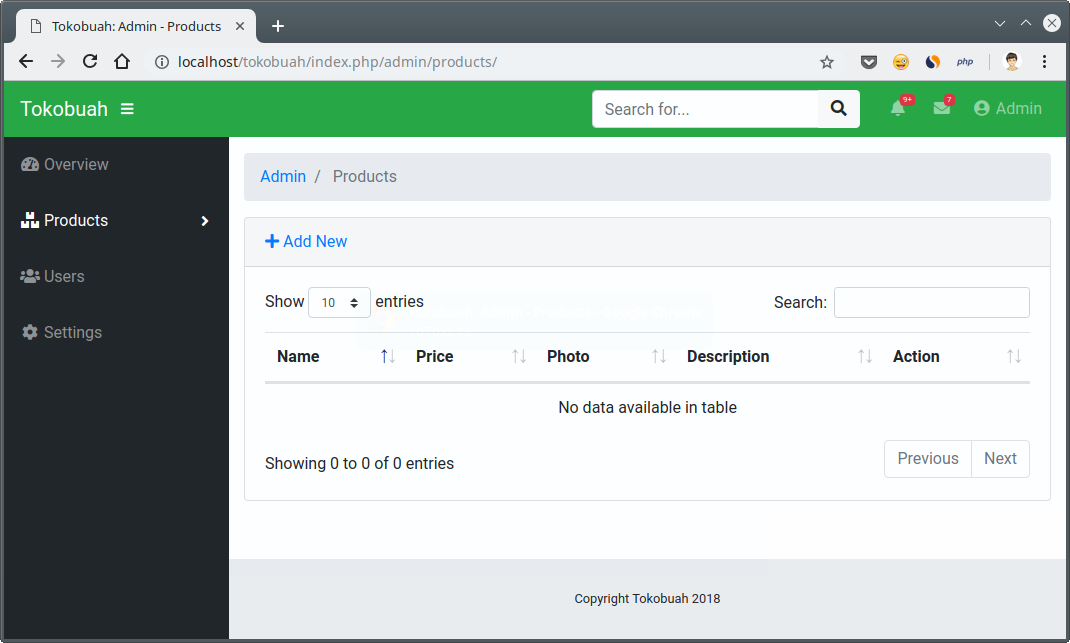The screenshot displays an administrative interface for a website called Tokobuwa. At the top of the page, the browser's address bar reads "localhost/Tokobuwa/index.php/admin/products/". The browser tab is labeled "Tokobuwa Admin - Products". On the right side of the top bar, icons are displayed, including a happy face (smiley face) icon, an orange and black PHP symbol, and a generic profile picture icon. 

The upper left corner features a black bar containing an 'X' button and two navigation arrows. Directly below, a green bar displays the site name "Tokobuwa" adjacent to a search bar labeled "Search for...". Nearby are additional icons including a bell (notification) icon and an envelope (message) icon along with the identifier "admin".

On the left side of the screen, a vertical black menu lists options such as Overview, Products, Users, and Settings. The main content area, which is white, is titled "Admin Products" with an option to "Add New". Below this, there is a table setup for displaying product details with columns for "Name", "Price", "Photo", "Description", and "Action". The table header includes options to show 10 entries at a time and a currently empty search box.

At the bottom of the table, a message states "No data available in table" indicating that there are no entries to display. It also mentions "showing 0 to 0 of 0 entries", with navigation buttons for "Previous" and "Next" that are currently inactive. The footer at the bottom of the page reads "Copyright Tokobuwa 2018".